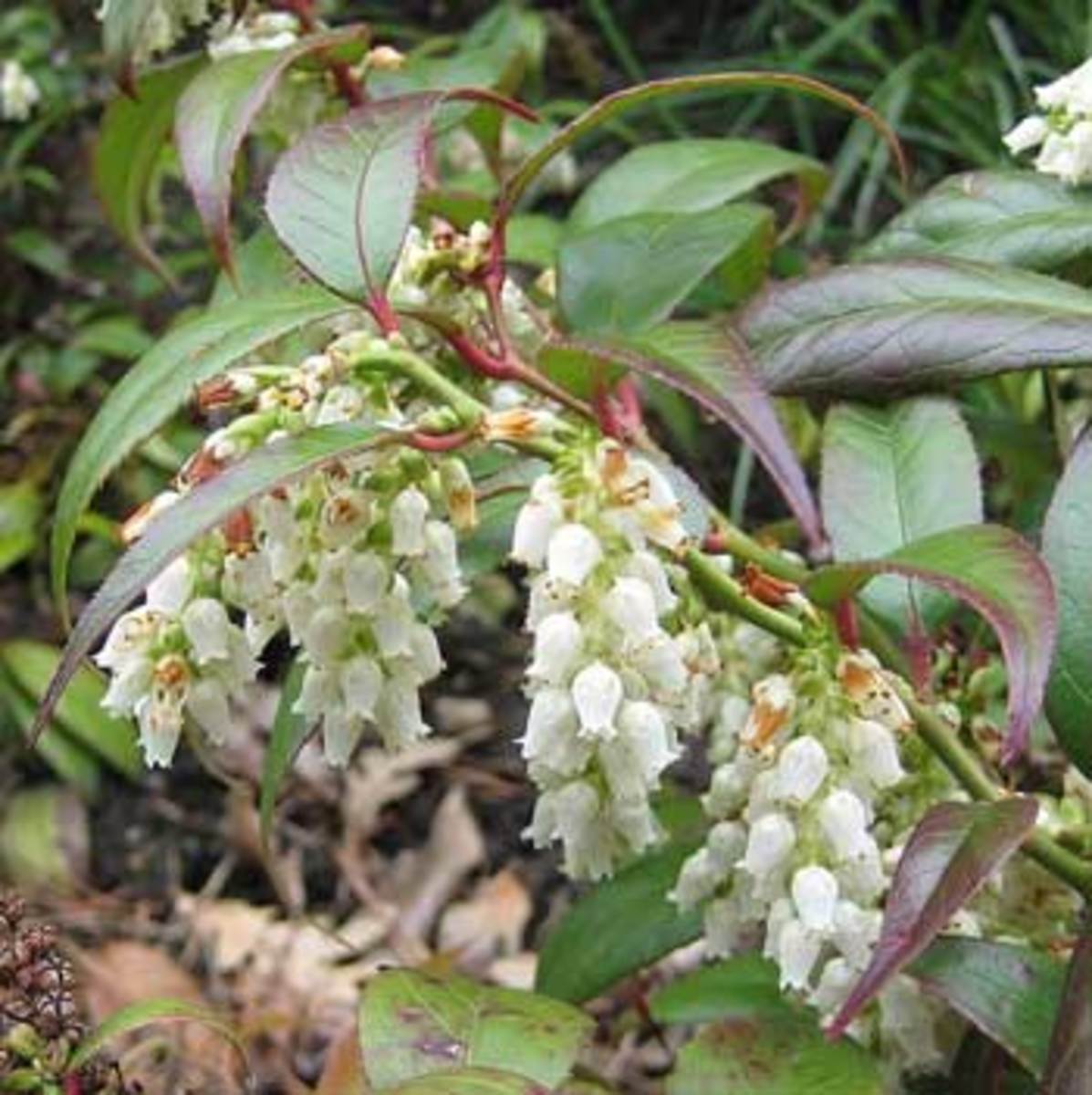This is a captivating close-up nature photograph of a flowering plant adorned with clusters of delicate, white, bell-shaped flowers. Each individual flower, numbering around a dozen to fifteen per cluster, dangles gracefully from a series of stems, giving the impression of miniature white bells or perhaps white Pac-Man ghosts due to their shape. These blossoms have a scalloped edge that adds to their fragile beauty. The plant itself boasts a robust, bright green central stem, from which all these flowering stems emerge. Surrounding the flowers are long, pointed leaves that feature an appealing interplay of green and deep purple, particularly accentuated along the veins and edges of the leaves. Some leaves exhibit tinges of red toward the edges and down the spine, adding vibrant splashes of color. The photograph appears to have been taken during the daytime and also captures the natural ground environment with some brown, fallen leaves scattered among the greens. The entire composition exudes a serene, almost ethereal charm, making it a picture-perfect moment one might encounter during a leisurely hike.